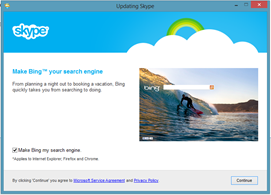This image is a screenshot of a window displaying instructions for updating Skype. It features a blue Windows interface, outlined in a medium blue border. At the top of the window, there are icons for minimizing, maximizing, and closing the screen, represented by the standard Windows controls: a dash, a square, and a red X, respectively.

In the center of the window, black text reads "Updating Skype." The top section of the window has a baby blue bar featuring the Skype logo on the upper left. On the right side of this bar, there are cloud imagery and a green and yellow arch, adding a touch of color and design to the interface.

Below this bar, the background transitions to white, adorned with blue and black text as well as a photograph. On the left side of the white background, blue text instructs, "Make Bing your search engine." Underneath, in somewhat out-of-focus black text, the message reads, "From planning a night out to booking a vacation, Bing quickly takes you from searching to doing." 

Adjacent to this text is a vivid photograph of a surfer riding within the curve of a breaking wave, with the Bing search bar superimposed on it. Below this image is an option reading "Make Bing my search engine," which includes a checkbox for users to select.

At the bottom of the window, there is a gray rectangle that houses navigational elements, including a prominent "Continue" button located at the bottom right corner.